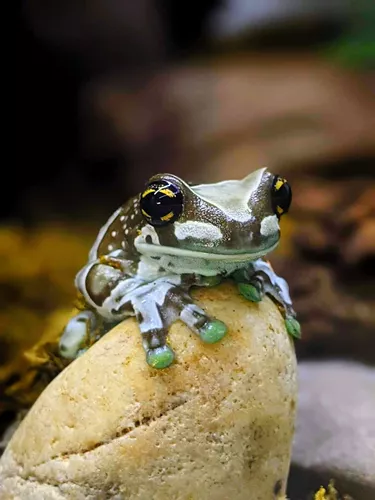This is an up-close photograph of a beautiful and colorful little tree frog, perched squarely on a yellow-tinged white rock with subtle etchings. The frog, which looks both slimy and endearing, has an intricate speckled pattern of olive green and brown on its body. It boasts striking bright green fingertips and speckled legs similar to its face, with green and yellow dot accents. Its large eyes are a captivating mix of black and gold, outlined with four yellow stripes that form a roughly circular pattern, giving an impression of a wide, almost smiling expression. The frog gazes directly into the camera, seemingly inviting interaction. The background is deeply out of focus, emphasizing the frog and suggesting a natural habitat without providing specific details.